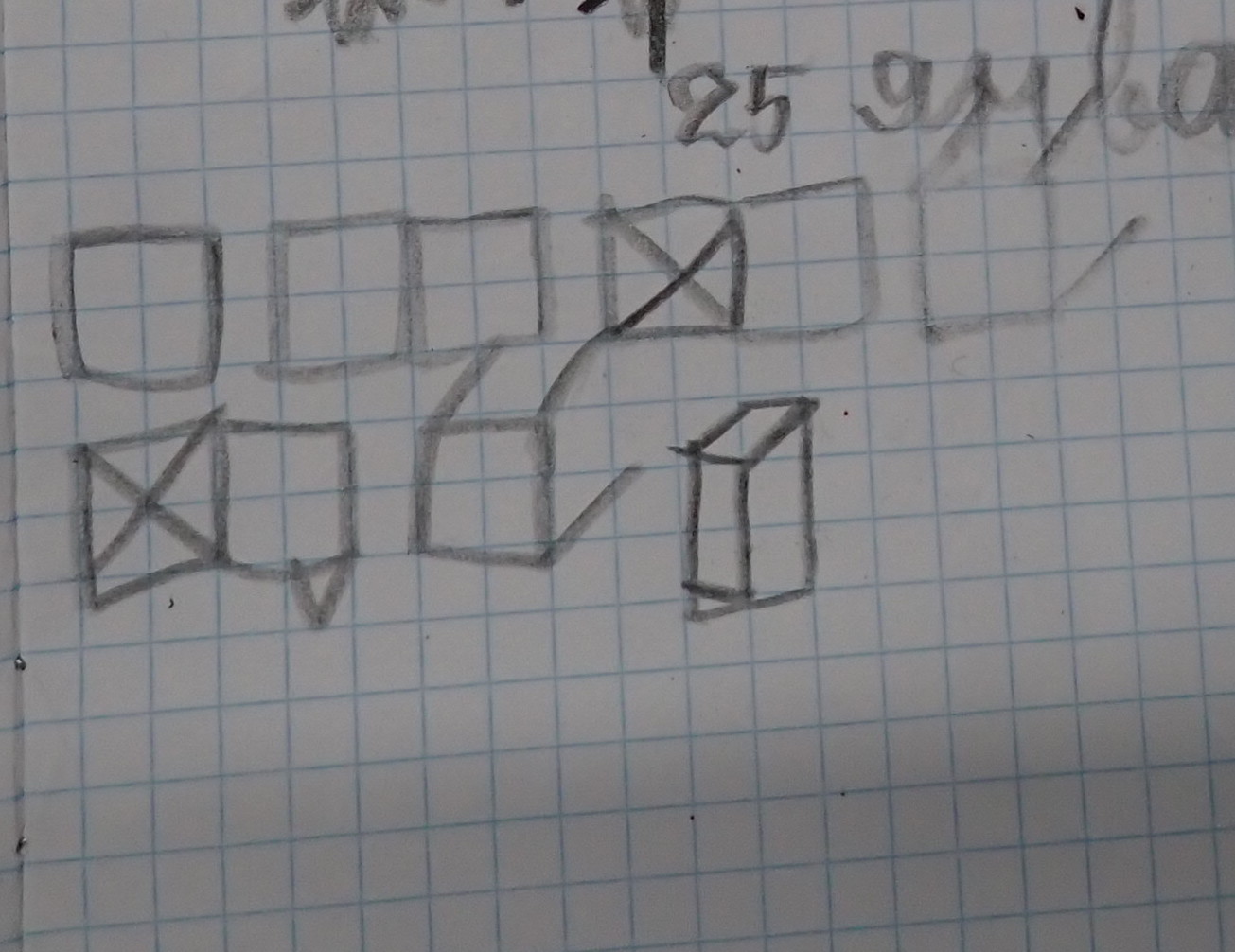A portion of a piece of white graph paper with light blue lines is covered with various hand-drawn shapes and numbers. Among the drawings, there are several squares, some of which contain an X in the center. Each of the circles depicted on the paper encloses four squares of the grid. On one part of the paper, some squares have triangles extending from their sides.

Additionally, the drawings include images that resemble furniture. For instance, one sketch appears to be a table with four legs, and there are two images that look like tables. Another drawing resembles a podium, the kind used for giving speeches. Amidst the doodles, there's some handwriting, possibly the name "Julia," although it's partially obscured by other sketches.

Most of the drawings appear to be made with a black crayon, giving them a range of shades from light gray to darker tones. The overall effect is a collage of geometric shapes and objects, rendered in a somewhat messy but intriguing arrangement.